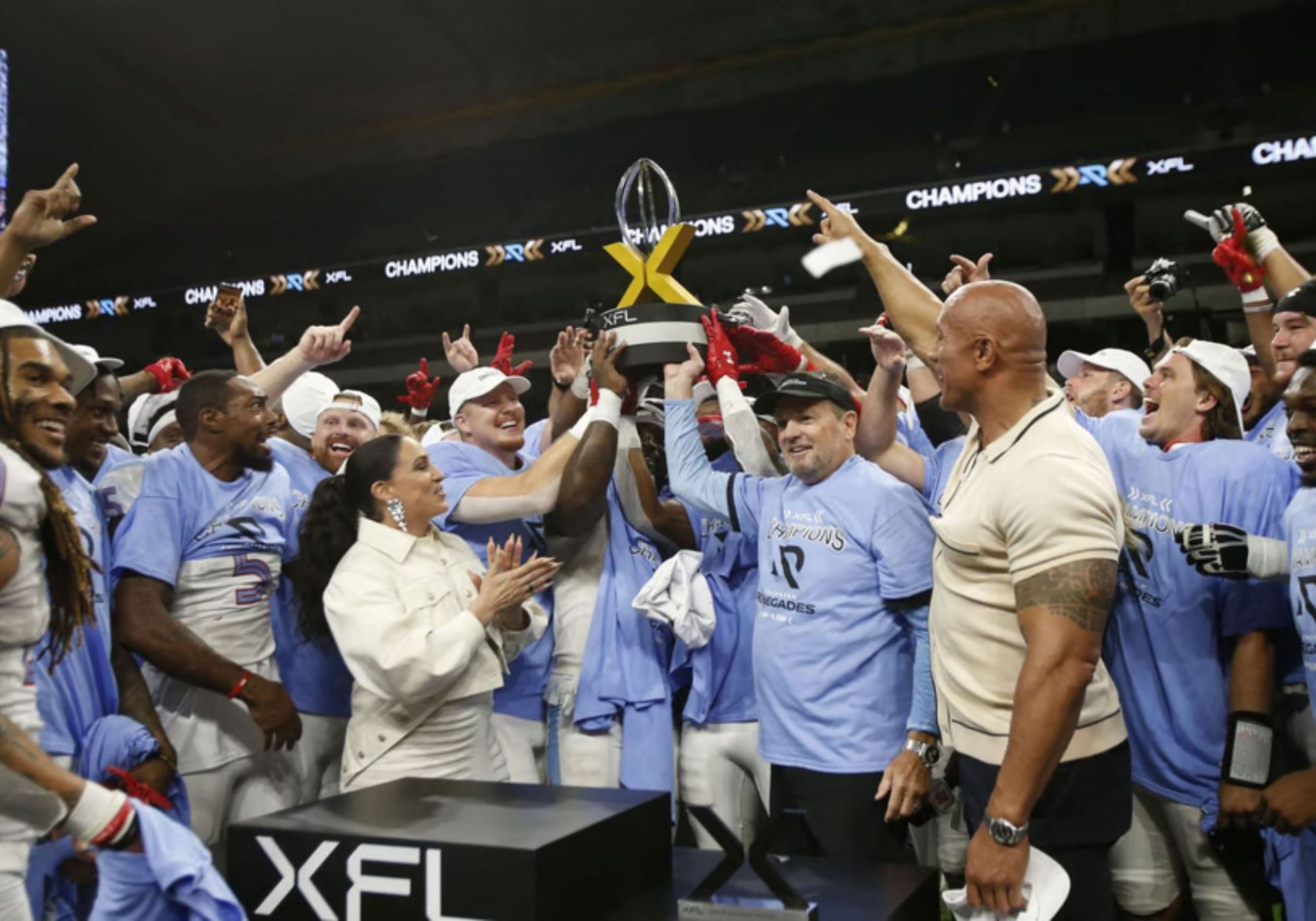This photograph captures the jubilant celebration of the XFL championship trophy ceremony. The focal point is the XFL trophy, prominently featuring a silver football and a large X, hoisted high by the ecstatic players and coach, all dressed in blue t-shirts with white hats indicating their championship status. To the right, Dwayne "The Rock" Johnson gestures upward, directing attention to the trophy. Additionally, a woman clad in a stylish white jacket and dress is seen joining the celebration with applause. The podium in the foreground bears the XFL logo, anchoring the scene. A sense of triumph fills the air as fists and fingers point upwards, embodying the "We're number one" sentiment. Background elements include the upper level of the stadium adorned with a ticker that repeatedly declares "Champions XFL." The entire scene is a vibrant tableau of smiles, cheers, and overarching excitement, making the moment unforgettable.